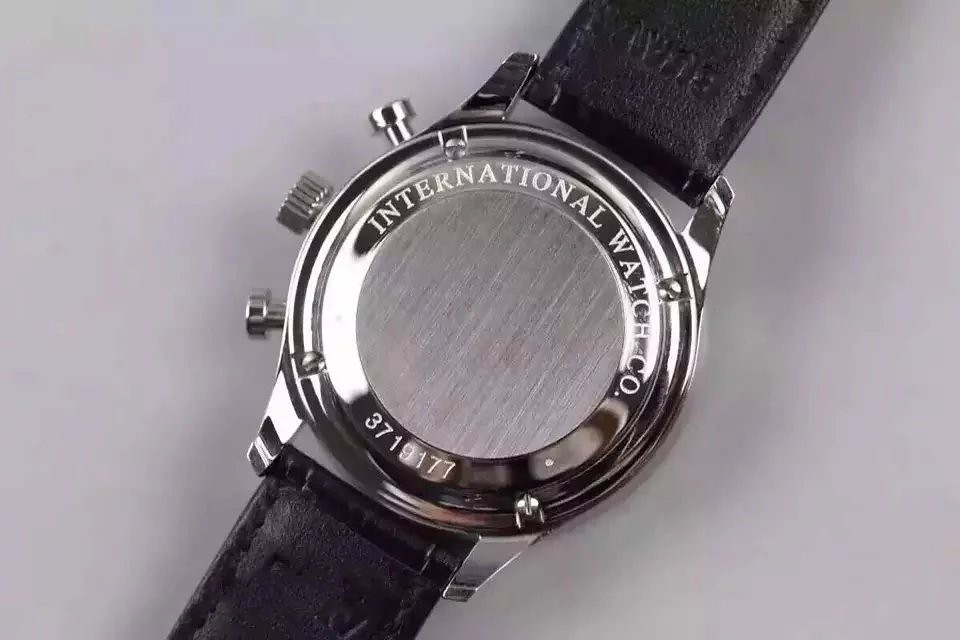A close-up photograph captures the intricacies of a wristwatch's backside, highlighting its meticulous design. The image focuses on the stainless steel back of the watch, where the dial itself is not visible. Engraved on the upper arc surrounding the case is the text "International Watch Co." Below, on the lower arc, the serial number "3719177" is etched into the metal. Flanking the sides of the watch case, three tiny knobs are observable, likely used for adjusting the time. The band, made of black leather, is partially visible at both the top and bottom of the frame. The entire scene is set against a stark white background, accentuating the subtle shadow cast by the watch, adding depth to this detailed composition.